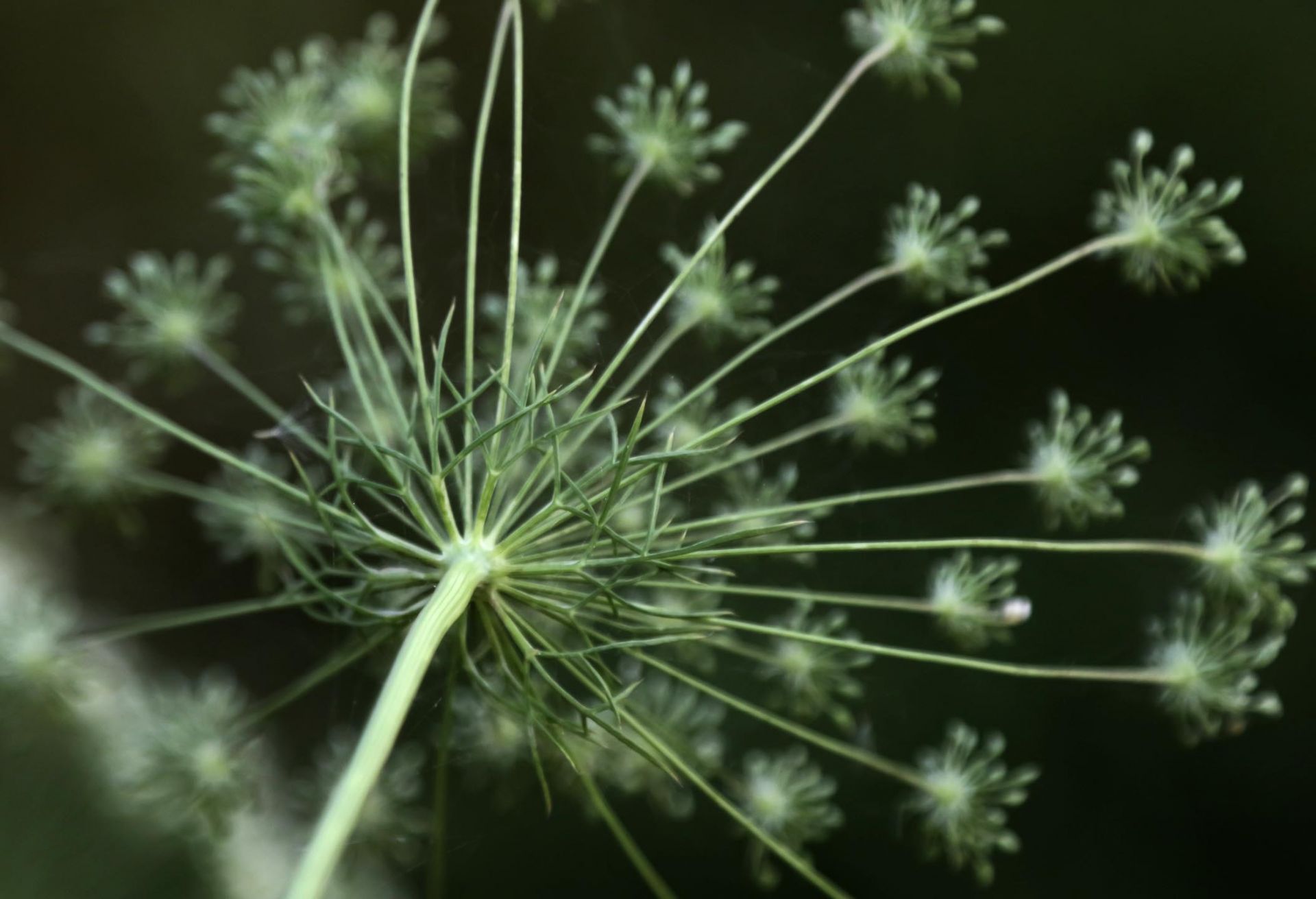This image features an intricate close-up of a plant resembling a dandelion, set against a pitch-black or very dark blue background. Prominently displayed is a light green stem, positioned diagonally at an approximate 20-degree angle towards the bottom left. Emerging from this stem are thorny, zigzagging shoots in varying shades of green, sprawling out in multiple directions. Additionally, delicate arms branch off the main stem, each ending in small budding points that resemble miniature green fireworks, further adding to the intricacy and beauty of the plant's structure. The backdrop is completely dark, offering no contextual hints of the location, and keeping the focus entirely on the detailed and vivid portrayal of the dandelion-like plant.